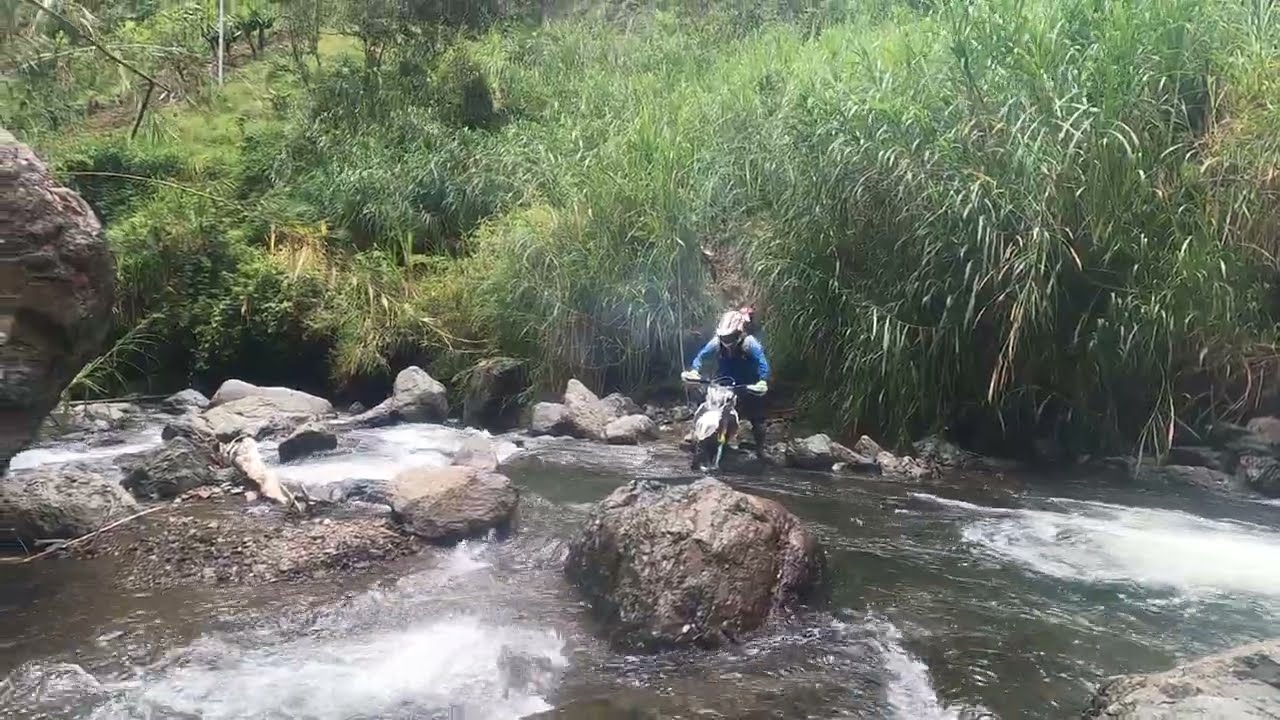In this landscape photograph, a man on a white dirt bike is captured at the edge of a rocky stream, seemingly contemplating his next move. The rider, dressed in a blue long-sleeve shirt and wearing a white and black helmet, is positioned centrally, with his hands firmly on the handlebars. The scene features a rocky stream running horizontally across the bottom half of the image. The stream is dotted with medium and large rocks, challenging the rider's path. The surroundings are lush and heavily vegetated, with dense foliage, towering trees, and thick, bushy grass filling the top half of the frame. The rider appears to have just exited a forested trail and now faces the decision of whether to cross the stream or turn back. The image conveys a sense of adventure and the rugged terrain encountered while dirt biking in a forested area.